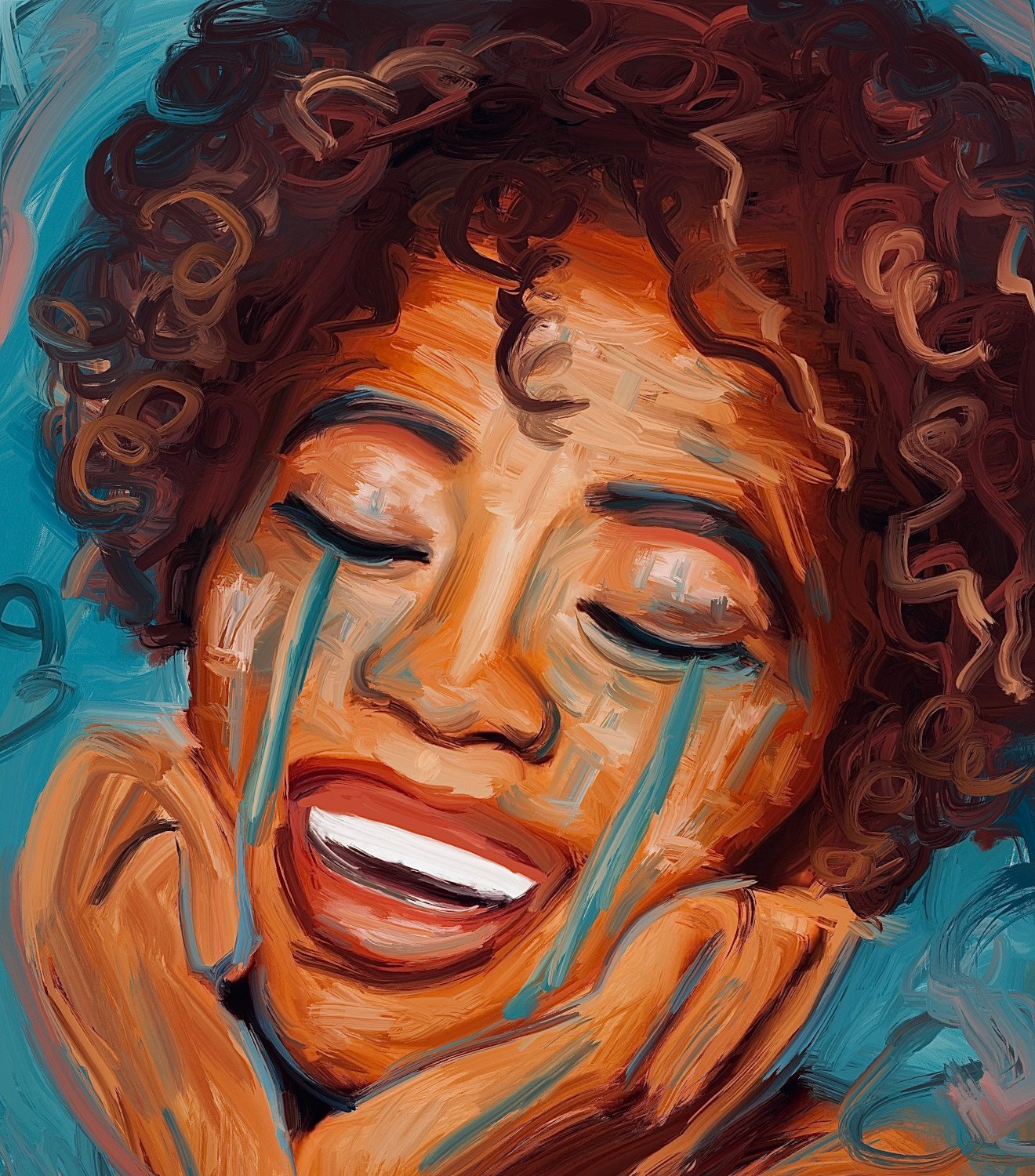The image is a digital abstract portrait of an African-American woman in a surrealistic style. The woman resembles Whitney Houston and has curly dark brown and black hair framing her face. Her eyes are closed, and streams of bluish-teal tears, possibly streaks of makeup, flow down her cheeks. Her orange-yellow face contrasts with her thick brownish-red lips, parted to reveal her bright white teeth. The portrait is set against an aqua blue background, interspersed with pink and darker blue swatches and lines. The woman's head is tilted to the right, with her chin and cheek cradled in her hands. The expressive and evocative details of the portrait create a powerful visual impact.